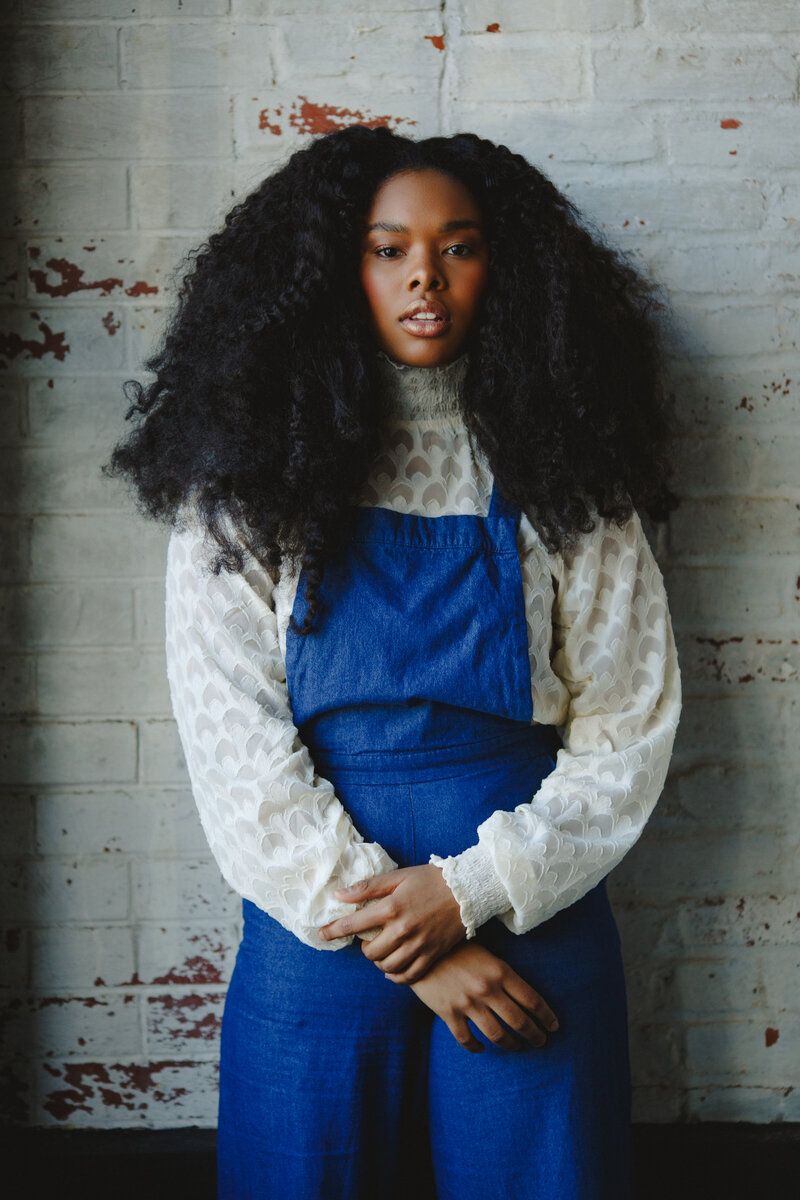This vertically-aligned rectangular image features a woman standing against a stained white brick wall. Visible from her knees up, the wall behind her shows worn white paint with scattered orange and red stains, and some brown and solid black marks near the bottom. The woman has a dark complexion and voluminous, curly black hair parted in the middle, spilling over her shoulders on either side. Her expression is neutral with her mouth slightly open, revealing her teeth. She is dressed in a blue denim jumper over a long-sleeve white shirt, patterned with curved lines and featuring a mock neck style. Her sleeves have elastic bands at the wrists. Her hands are crossed in front of her waist, with her left hand resting over her right wrist. The composition captures the rich textures of both her attire and the background, providing a contrast between her polished look and the distressed wall behind her.